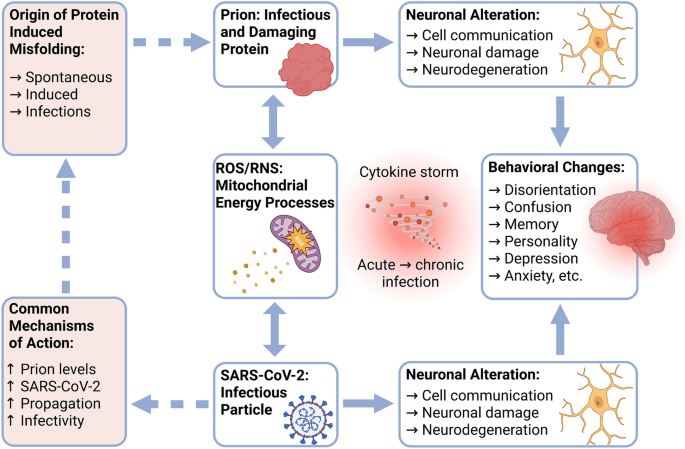The image is a detailed flowchart depicting the cascade of events leading to neurodegeneration and behavioral changes due to protein misfolding and infections, including SARS-CoV-2. The flowchart begins with a pinkish box labeled "Origin of Protein-Induced Misfolding: Spontaneous, Induced, Infections." An arrow leads to a box labeled "Prion: Infectious and Damaging Protein," illustrated with a piece of protein. From there, it continues to "Neuronal Alteration, Cell Communication, Neuronal Damage, Neurodegeneration," depicted with yellow nerves. This stage leads downward to a box showing a brain with a red center, labeled "Behavioral Changes: Disorientation, Confusion, Memory, Personality, Depression, Anxiety, etc."

This central "Behavioral Changes" box is flanked by two similar boxes on the top and bottom, both labeled "Neuronal Alteration, Cell Communication, Neuronal Damage, Neurodegeneration," also illustrated with neurons. To the left of the central box is a representation of a cytokine storm, depicted as a cyclone with microbes, labeled "Cytokine Storm: Acute to Chronic Infection." Above it is a box labeled "ROS/RNS: Mitochondrial Energy Processes," showing a purple cell amidst dots symbolizing microbes. Below this, the box labeled "SARS-CoV-2: Infectious Particle" links to the rest of the chart with an arrow.

To the left of the SARS-CoV-2 box is another labeled "Common Mechanisms of Action: Prion Levels, SARS-CoV-2, Propagation, Infectivity," illustrating connections with arrows. This comprehensive diagram visually represents the step-by-step progression from initial protein misfolding to complex neurodegenerative changes, interlinking with infectious mechanisms like SARS-CoV-2.